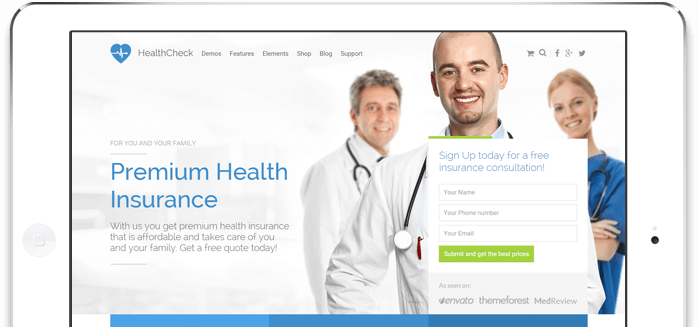The image depicts a detailed screenshot in landscape orientation, resembling a smartphone turned on its side, indicated by its rounded corners and the presence of a black dot on the right side, likely functioning as the power button. On the left side, there's an opaque gray circle containing a square, presumably the camera.

The main content displayed is a health insurance website captured within a black-bordered rectangle. At the bottom of this rectangle, a blue line is segmented into three shades: transitioning from light blue to medium blue, slate blue, and finally a darker blue.

In the top left corner, a blue heart icon is displayed, incorporating a graph typically used to measure heart rhythms in medical settings. This is labeled as "Health Check." Directly beneath are six menu options: Demos, Features, Elements, Shop (illegibly tiny), an unidentified entry, and Support.

Occupying the right side of the screenshot is a photographic image featuring three healthcare workers. In the foreground stands a jovial, young, balding physician with a broad smile, bushy black eyebrows, Caucasian complexion, adorned in a white lab coat with a stethoscope around his neck. Overlaying this individual is a white square that prompts viewers to "Sign up today for a free insurance consultation," with fields for Name, Phone Number, Email, and a green button labeled "Submit and Get a Free Quote."

Standing behind him are two additional healthcare professionals: one with salt-and-pepper hair reminiscent of Hugh Grant, clad similarly in a lab coat and stethoscope, and a young woman with reddish hair tied back, dressed in blue scrubs and also sporting a stethoscope, her arms folded confidently. Above her head is a row of five small icons: a shopping cart, a search magnifying glass, the Facebook "F," possibly the Google "G," and the Twitter bird.

To the left of the photographic illustration, prominently displayed in blue large letters, it states "Premium Health Insurance." Below, in smaller gray letters, it advertises, "With us you get premium health insurance that is affordable and takes care of you and your family. Get a free quote today."